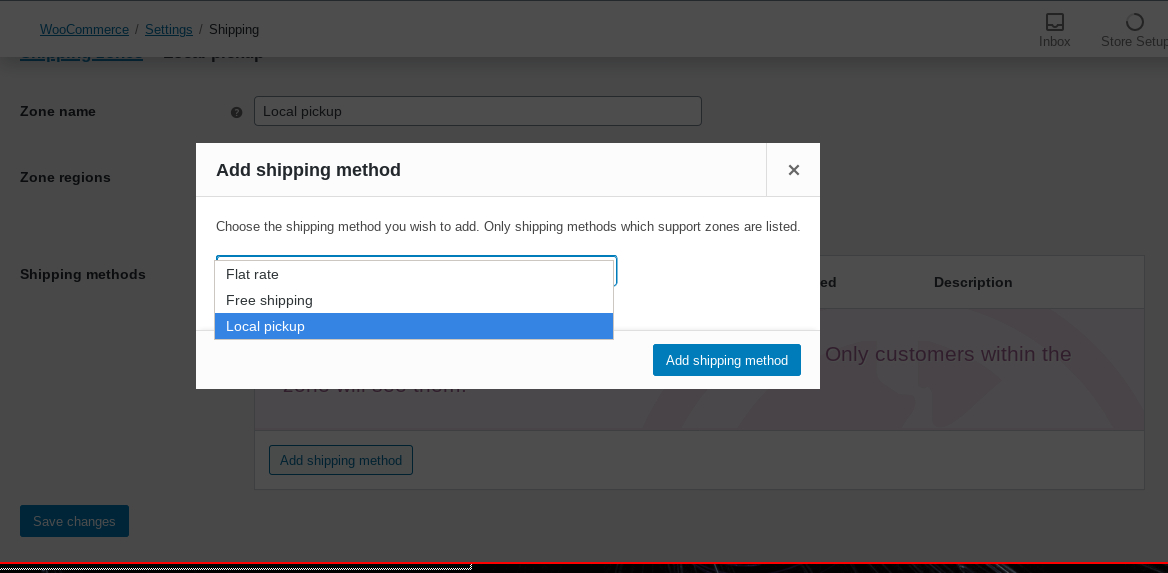The image is a detailed screenshot of the WooCommerce interface, focusing on the settings for configuring shipping methods. A prominent red bar at the bottom suggests the presence of a video, though it could also be a part of the screenshot itself. The main section of the page is under the shipping settings tab, where a user is choosing a shipping method for their online store.

At the top, key elements include a zone name labeled "local pickup" and a zone region, which is partially obscured by a pop-up. The configuration interface displays a clear instruction stating, "Choose the shipping method you wish to add. Only shipping methods which support zones are listed in this case." Below this, options are presented in a drop-down menu, consisting of "Flat rate," "Free shipping," and "Local pickup." The selected option is highlighted by a blue button, indicating the user’s current choice.

In addition to the primary shipping settings, the interface features an inbox and store settings icons located at the top right corner, allowing the user to manage communications and store configurations efficiently. The user is provided with a comprehensive section to input detailed information regarding the shipping options, aimed at facilitating prospective buyers in making informed purchasing decisions. Despite the central pop-up partially obstructing some on-screen elements, the overall intent and functional aspects of the WooCommerce shipping settings are clearly depicted.